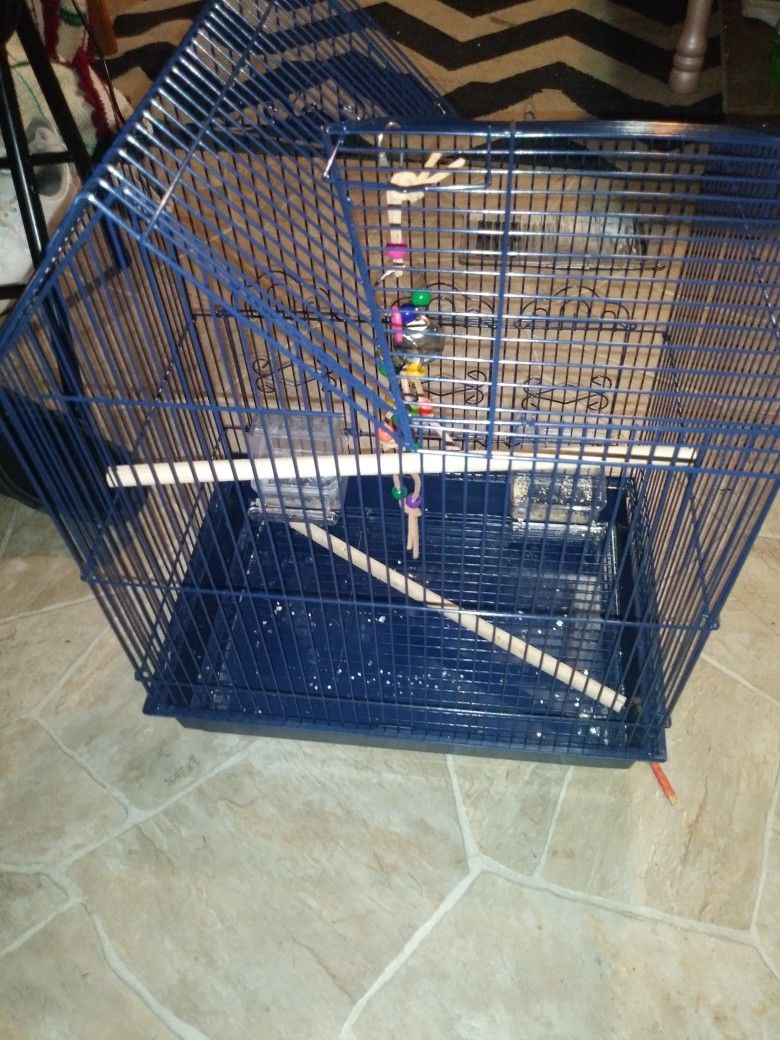The photograph depicts a large, unusual-looking bird cage made of blue metal wire, placed on an irregular, tannish-beige tile floor. The bird cage features a distinctive design with a steep triangular roof on the left side transitioning to a flat roof on the right, adding to its unconventional appearance. Despite its spacious and deep interior, no birds are present; instead, a colorful bird toy hangs from the top. This multicolored toy, adorned with blue, green, yellow, pink, red, purple, and orange beads, features a leather tie and possibly a bell or mirror, alongside bits of rope.

Within the cage, a whimsical scene unfolds with figures resembling acrobats from a circus. These brightly dressed figures form a human pyramid, starting from the very top and cascading down to a person standing at the bottom, seemingly supporting the entire assemblage on his shoulders. Additionally, the cage contains two perches—one arranged horizontally and another resting on the cage floor—along with a mostly empty food container and scattered seed shells. 

In the backdrop, a black-and-white zigzag patterned rug can be seen, and the setting suggests that the cage is situated in a living room or foyer. The base of the bird cage is a solid blue rectangular shape, completing the unusual and detailed scene displayed in the photograph.